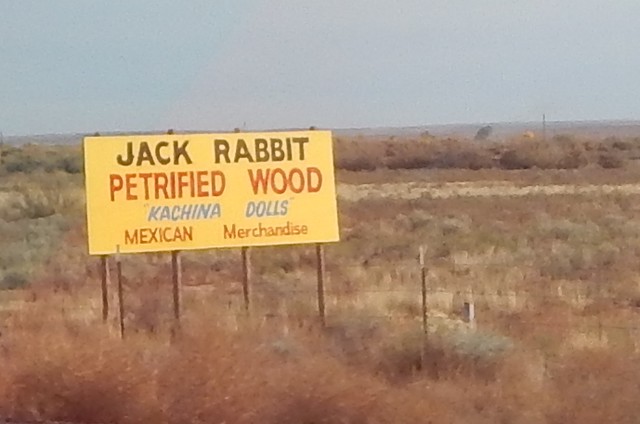The image depicts a seemingly vintage landscape photograph taken alongside a road in a desert-like, southwestern area of Mexico. Dominating the foreground is a handmade yellow sign, supported by four round wooden poles resembling telephone poles. The weathered sign, which has a rustic, old-world character, advertises "Jack Rabbit Petrified Wood" in brown paint, "Kachina Dolls" in blue, and "Mexican Merchandise" in a lighter brown. Spanning the scene is an expanse of prickly, overgrown scrub brush, interspersed with hints of green cacti, and possibly a touch of wild red brush near the sign. A barbed wire fence with metal posts runs in front of the sign, further emphasizing the rugged, untamed nature of the landscape. The horizon showcases a line of darker blue mountains against a light blue sky, enhancing the vastness and arid beauty of the scene.